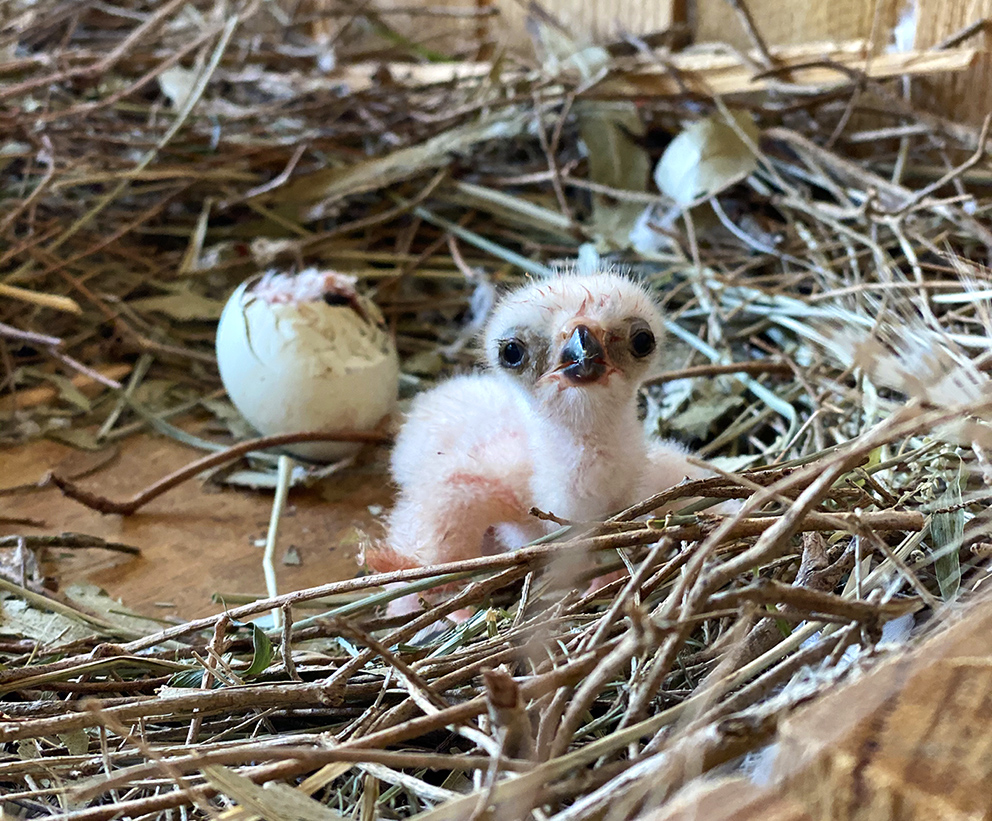The image is a detailed, color photograph of a newly hatched baby eagle, prominently positioned at the center. The eagle, covered predominantly in white downy feathers, has areas where its wet fur reveals pink stains, indicative of its recent emergence from the egg. The hatchling sports wide-set black eyes and a distinct, triangular black beak, gazing directly at the viewer with its head slightly raised. Situated on a brown surface that forms the nest, the scene is encircled by numerous large tree branches and small twigs. To the left of the fledgling, a cracked white egg shell, from which it presumably hatched, is slightly tucked into the background, contributing to the naturalistic setting. The composition evokes a sense of raw realism, capturing the tender moment within a nest, possibly deep in the wild or a protected environment.